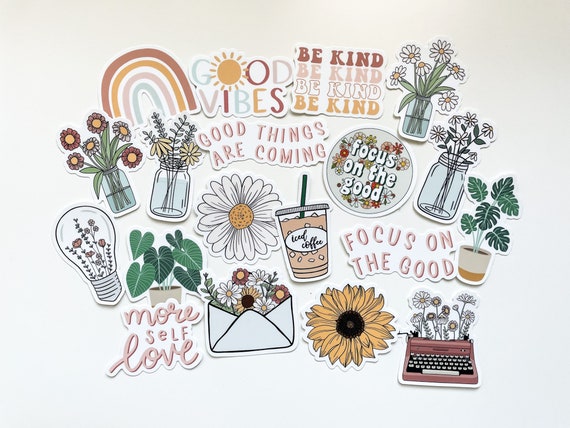This image showcases a diverse collection of colorful stickers and decals arranged on a grey background. Central to the design is a vibrant "Good Vibes" sticker, with the 'O' cleverly depicted as a sun, utilizing a color scheme of burnt orange, rusty red, light pink, blue, and white. Among these, a striking rainbow sticker with hues of brown, orange, pink, and green catches the eye. Another prominent sticker repeats the phrase "Be kind" in four different colors.

In addition to motivational messages, the scene is adorned with botanical imagery, including clear glass mason jars filled with white daisies and greenery, red flowers, and yellow and pink flowers. There’s a tan flower pot overflowing with green plants, and an array of other floral decals including sunflowers and daisies.

Further details include an iced coffee cup labeled "Seed coffee", a typewriter bursting with flowers, and a light bulb similarly filled with blooms. A sticker that reads "More self-love" and another with "Good things are coming" add to the positive affirmations scattered throughout. The design culminates with several decals bearing the phrase "Focus on the good" against various backdrops, emphasizing an uplifting, cohesive theme.